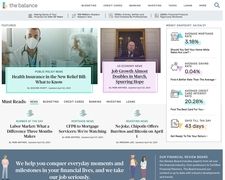The image appears to be a screenshot of a medical news article from a website that seems to be titled "The Balance," indicated by the light grey text at the top. The website interface has several unreadable tabs and a magnifying glass icon on the far right corner, likely for search purposes. Below this, there is a grey horizontal strip with some text that remains blurry and unreadable.

On the left side of the main content area is a photo of a doctor. He appears to be a man with tan skin, sporting very short, shaven hair. He is wearing a white surgical mask covering his mouth and nose, a stethoscope around his neck, and a white medical coat over light blue or green scrubs. Next to him, possibly accompanying him in the image, is a blurred figure who seems to be an elderly man.

To the right of this photo, there is a light green text box that looks like it contains an article, though the text is too blurry to read. Adjacent to this section, further to the right, there is another image. It appears to be a man standing on a stage behind a podium, possibly equipped with a microphone. The context is unclear due to the blurriness, but the word "job" can be seen within a light pink text box nearby.

Further to the right, statistical information is presented with figures such as 3.18%, 0.04%, 20.26%, and 45 days, although the finer print is unreadable. Above this information are light grey arrows, indicating more details that are also blurred.

At the bottom, there's a bluish-grey banner featuring animated images of three people, accompanied by some text that remains indistinct.